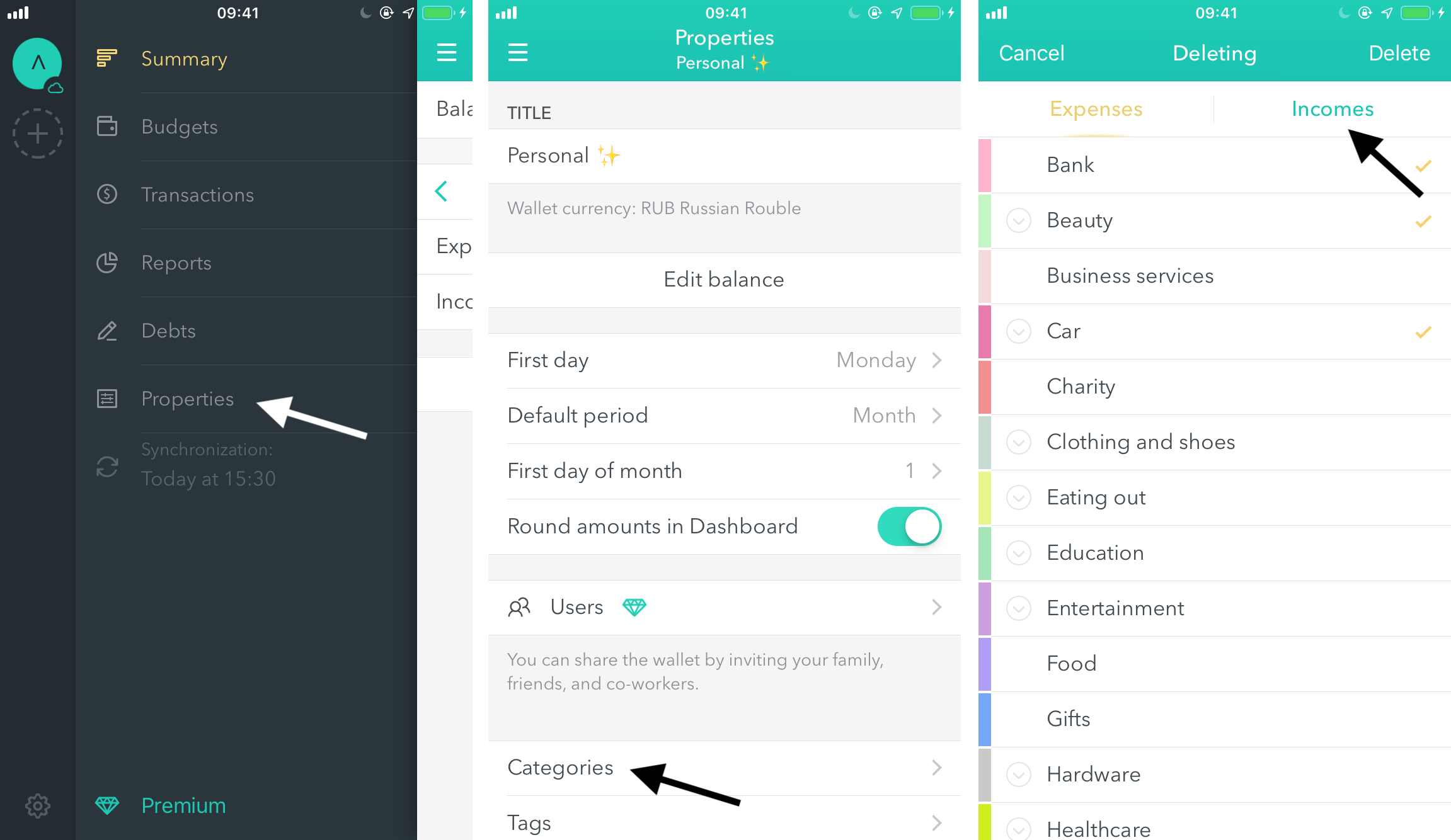**Screenshot Descriptions for Financial Management App**

1. **First Screenshot**: The background is black, displaying various financial management features. At the top, the time reads 15:30. Key elements include:
   - **Numerical Display**: "941" prominently in white.
   - **Highlighted Section**: "Summary" in yellow.
   - **Menu Options**: Budgets, Transactions, Reports, Debts, Properties, and Synchronization.
   - **Specific Focus**: A white arrow points towards "Properties."
   - **Footer Note**: "Premium" displayed at the bottom.

2. **Second Screenshot**: The background is white, detailing settings for a personal finance wallet. Time displayed is 09:41. Elements include:
   - **Heading**: "Title" labeled as "Personal Wallet."
   - **Financial Information**: Currency set to RUB (Russian Ruble), with options to edit the balance.
   - **Configuration Settings**: 
     - **Default Period**: Starts on Monday.
     - **Month Configuration**: Begins on the first day.
   - **Dashboard Settings**: "Round amounts in dashboard" toggle is turned on.
   - **Sharing Options**: Invite family, friends, and co-workers to collaborate on the wallet.
   - **Categories and Tags**: A black arrow points to "Categories."

3. **Third Screenshot**: Displays an overview of financial transactions with a time stamp of 09:41. On a predominantly white interface, key features include:
   - **Section Titles**: "Expenses" in orange and "Incomes" in green.
   - **Interactive Element**: A black arrow indicating "Incomes."
   - **Transactional Categories**: Highlighted items with check marks include Bank, Beauty, and Car under Expenses and Business Services.

These screenshots collectively demonstrate a user-friendly finance management app emphasizing ease of navigation and comprehensive functionality, from tracking budgets and transactions to customizing personal finance settings.